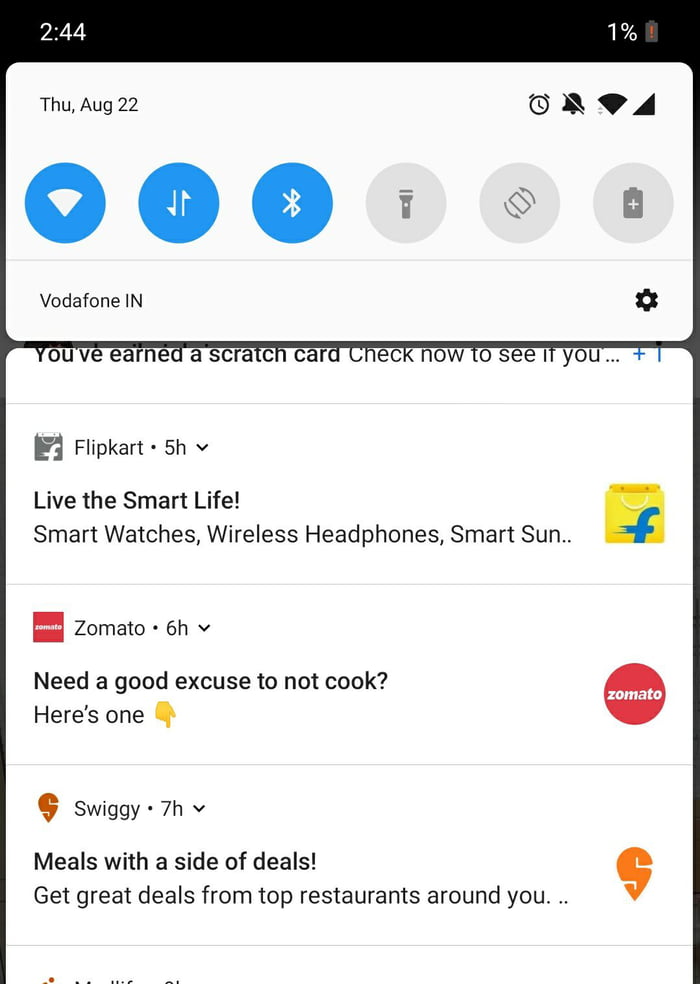This is a detailed screenshot from a person's cell phone. The top left of the screen displays the time as 2:54. At the top right, the battery indicator ominously shows only 1% remaining. Below the time, the date "Thursday, August 22nd" is visible, with icons for an alarm clock, volume, and Wi-Fi immediately below it. 

Directly under these, there is another row of icons for Wi-Fi, Bluetooth, flashlight, screen rotation, and battery status. Vodafone iN is the network provider shown.

Several notifications occupy the screen:
1. A Vodafone iN notification stating, "You've earned a scratch card. Click now to see more...".
2. A Flipkart notification indicating, "5 hours with the smart life. Smart watches, wireless headphones, smart sun...".
3. A Zomato notification from 6 hours ago reads, "Need a good excuse to not cook? Here's one ⬇️".
4. A Swiggy notification from 7 hours ago encourages, "Meals with a side of deals. Get great deals from top restaurants around you...".

The image is oriented vertically, being taller than it is wide. It contains no people, animals, birds, plants, flowers, trees, buildings, automobiles, motorcycles, or airplanes. The entire focus remains on the content displayed on the cell phone screen.